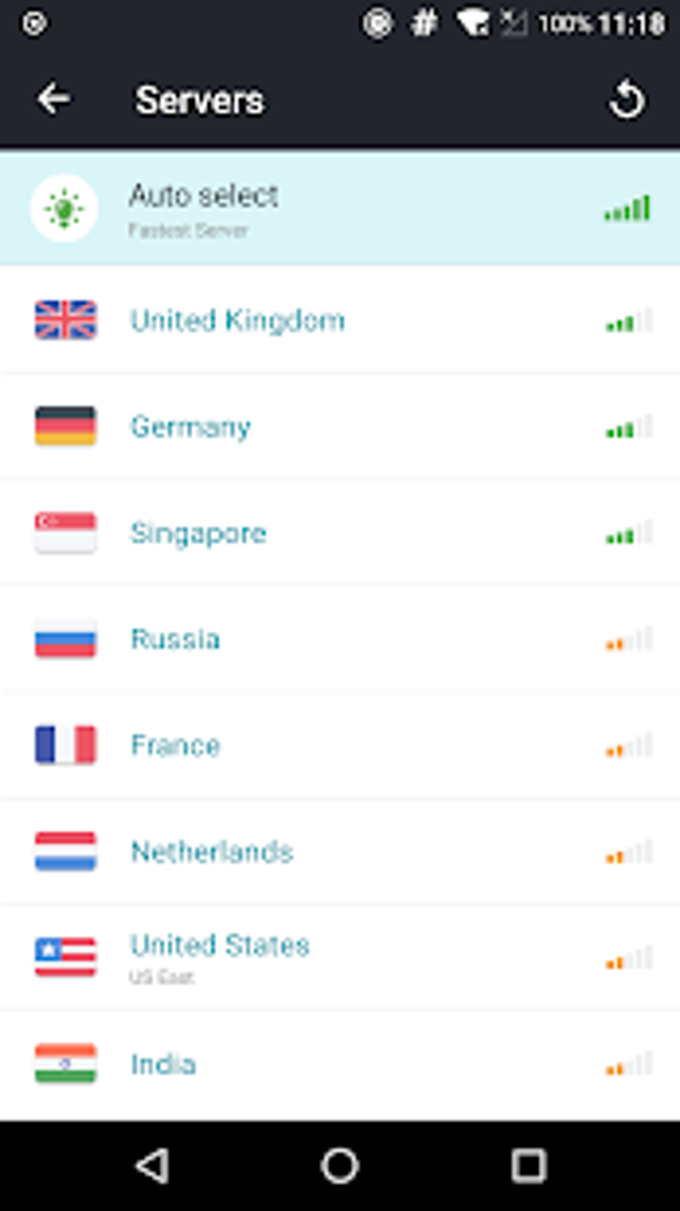This screenshot depicts a server selection interface. At the top, there's a black banner with the word "Servers" displayed in white font. To the left of the title is a white back button, and to the right, there is a white refresh button. Below this banner, a blue-highlighted row indicates that the "Auto-Select" option is currently selected. Within this row, a bright green light and a white circle are present, accompanied by the words "Auto-Select" in black text. Beneath this, in smaller font, it states "Fastest server."

On the right-hand side of the screen, a series of vertical bars represent server signal strength or performance, all colored in bright green, with the height of the bars increasing progressively. 

Further down, there's another row containing the words "United Kingdom" in blue text on a white background. To the left of this text, the flag of the United Kingdom is displayed, featuring a navy blue field with a red cross and a red X over it. To the right of this row, another set of vertical bars indicates the server's performance or connection strength, with three out of five bars highlighted in the same medium bright green color. This bar indicator is also consistent with the one in the top row.